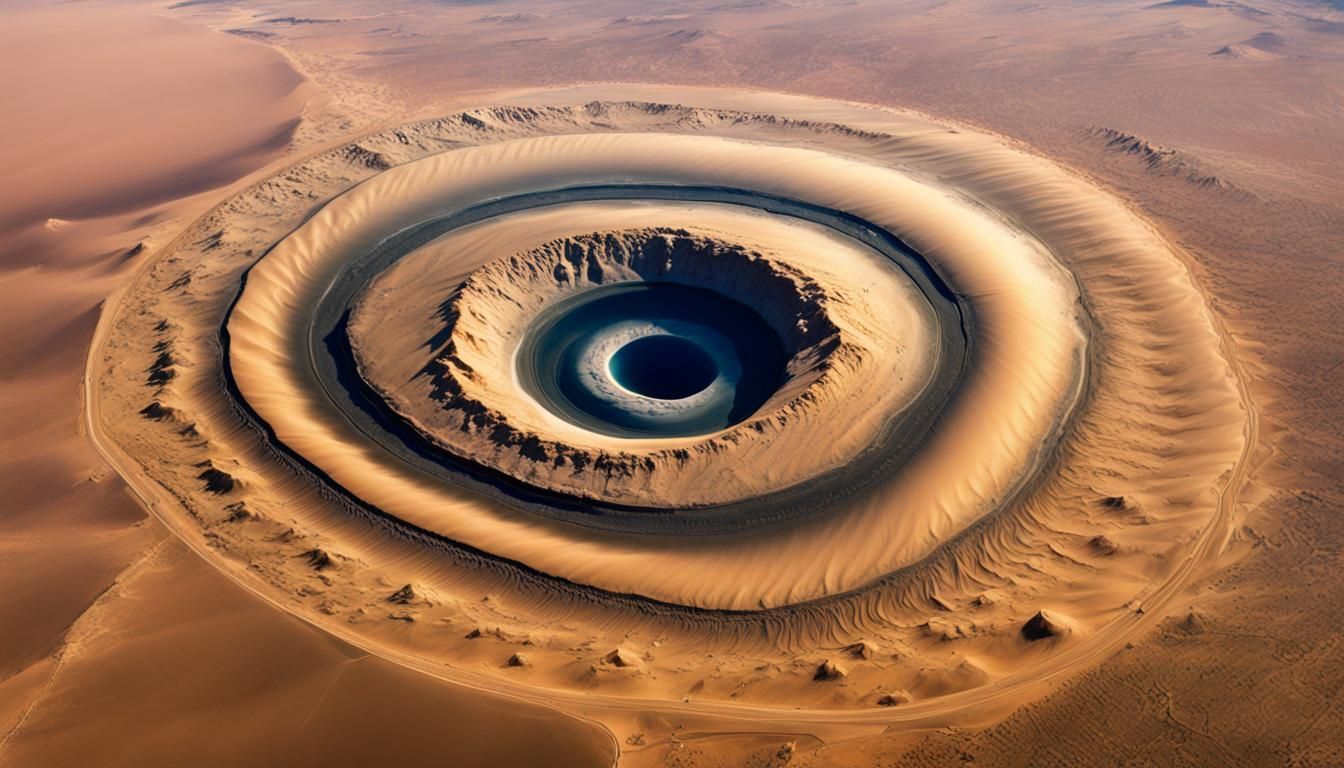The image, likely a photograph taken from the air or a computer-generated depiction, presents an intricate and artistic scene reminiscent of a desert landscape. Dominated by tan and yellow hues, the setting features natural-looking sand dunes with small outcroppings resembling hills and small mountains. At the center, a striking circular formation is carved into the sand. This formation consists of multiple concentric rings, alternating in color and shadow. The outermost rings are a blend of yellow and tan, gradually transitioning into darker shadowed areas as they approach the core. The very center features a recessed, dark well with a visually arresting, white-outlined shape resembling an iris, culminating in a profound black center. The scene is captured in bright daylight, enhancing the contrast and clarity of the formations and shadows, adding depth and a sunlit dimension to the surreal landscape.